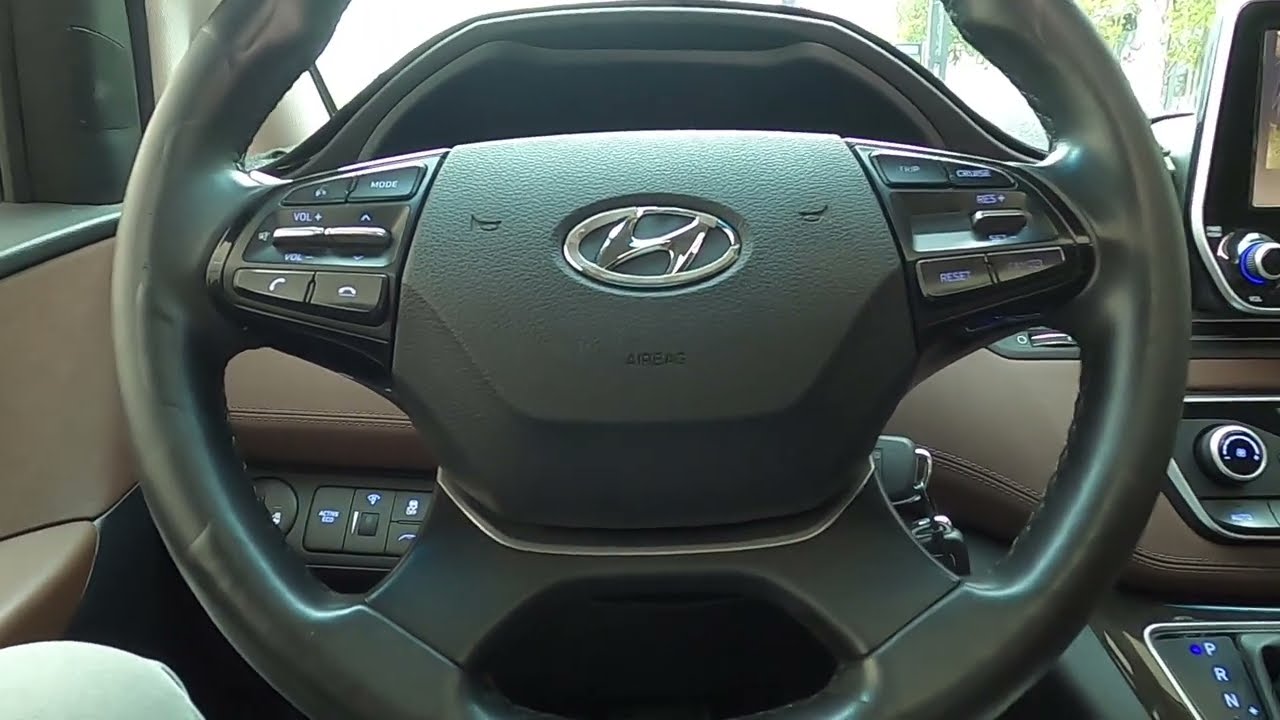This close-up image captures the detailed interior of a Hyundai sedan, focusing on the steering wheel prominently displaying the slanted Hyundai logo in the center. The steering wheel, made of black faux leather, is equipped with multiple functional buttons that manage volume control, phone calls, various modes, and possibly cruise control. It is held by four arms, and the top two arms house these buttons. The scene appears to be set during daylight hours, showcasing a well-lit interior with a hint of tan color. A digital display is partially visible to the right, indicating the car is parked, as evidenced by the blue dot next to the 'P' on the display. The car's interior, through the windshield, reveals a glimpse of trees outside, adding to the serene backdrop. The perspective suggests the viewer is sitting in the driver's seat, providing a detailed look at the clean and organized dashboard area and confirming the vehicle is a Hyundai.